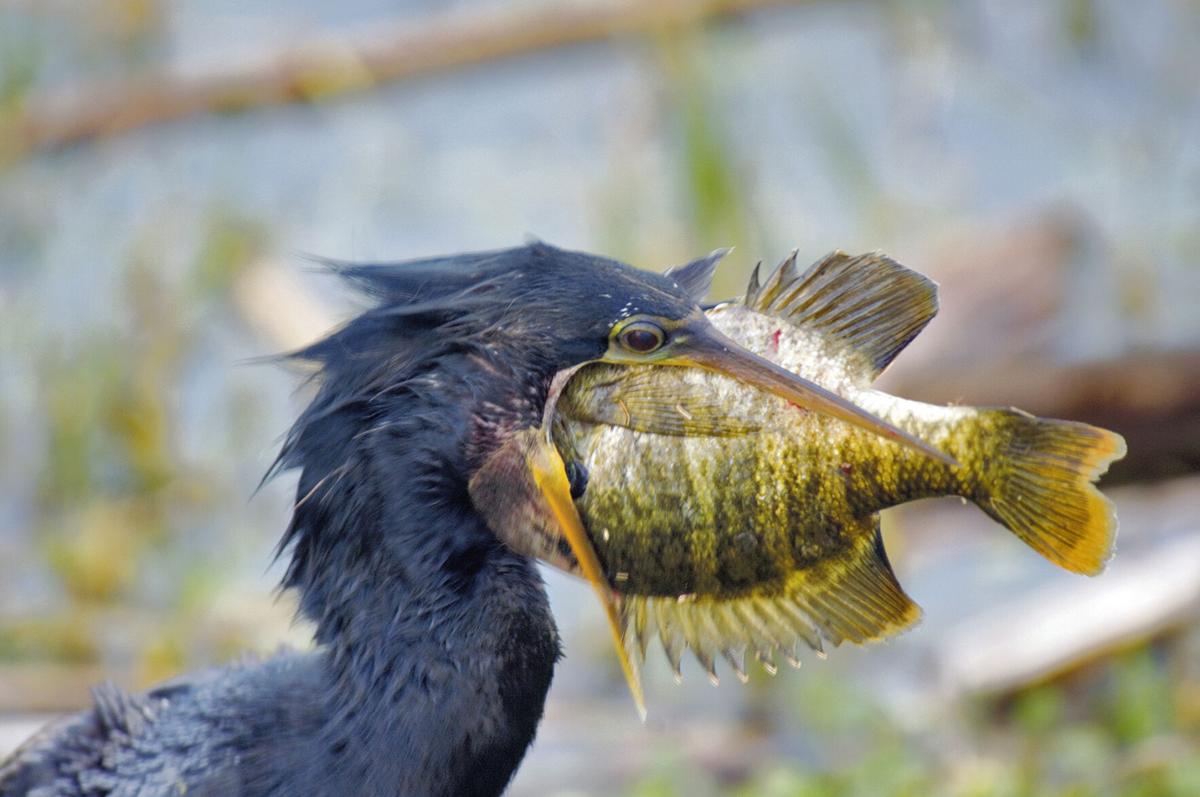In this vibrant daytime photograph, a determined black Cochrane bird, with wet feathers clinging together, is attempting to devour a sizeable fish that appears bigger than the bird's head. The bird's yellowish-black, long, and pointy beak is spread remarkably wide, almost as if its jaw is unhinged, in an effort to gulp down the fish. The fish itself, brightly colored in hues of yellow, brown, black, and with an orange tail, looks somewhat round and is adorned with sharp fins, suggesting it might be a perch or a carp. The bird’s keen black eyes, surrounded by a touch of yellow, reflect its predatory nature and excellent hunting skills. The background, while blurred, hints at a watery habitat with colors of brown, blue, yellow, and green, possibly including lily pads. There is no text within the image, allowing the focus to remain entirely on the dramatic struggle between the bird and its prey.